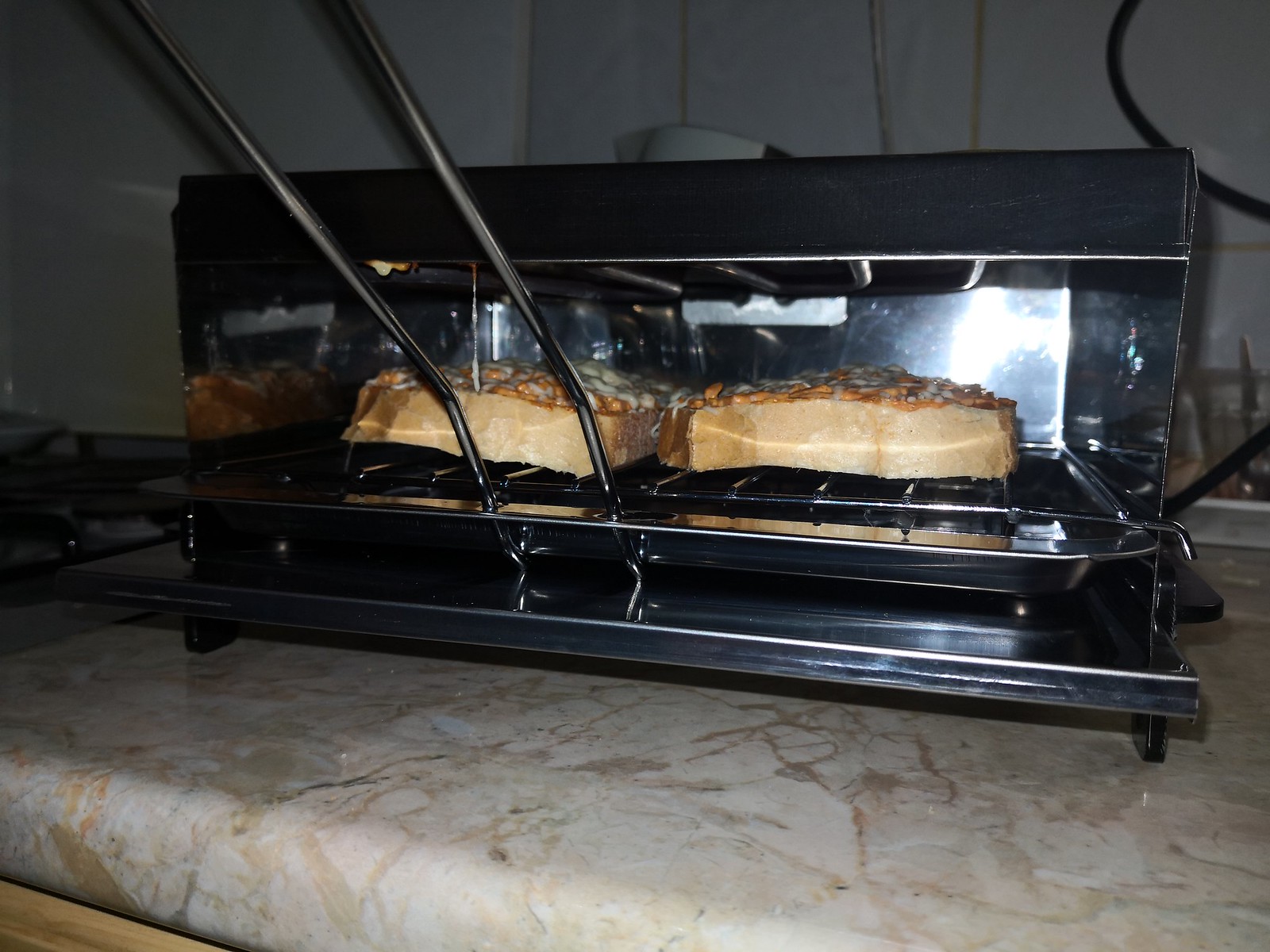In this detailed photograph taken in a horizontally-oriented kitchen, the main focus is a black and stainless steel toaster oven centered prominently on a countertop. The countertop appears to be marbled, predominantly beige with darker brown veining, imitating a granite surface. Inside the toaster oven, two pieces of bread with browned crusts sit on a silver tray featuring wire rods. The bread appears to be topped with melted cheese and a red sauce, possibly resembling pizza. The toaster oven door is open, revealing metal brackets and heating coils inside. The background showcases white tiled walls and a stovetop, with a dimly lit ambiance. A black cable extends from the wall into the toaster oven, adding to the kitchen scene's detailed complexity.